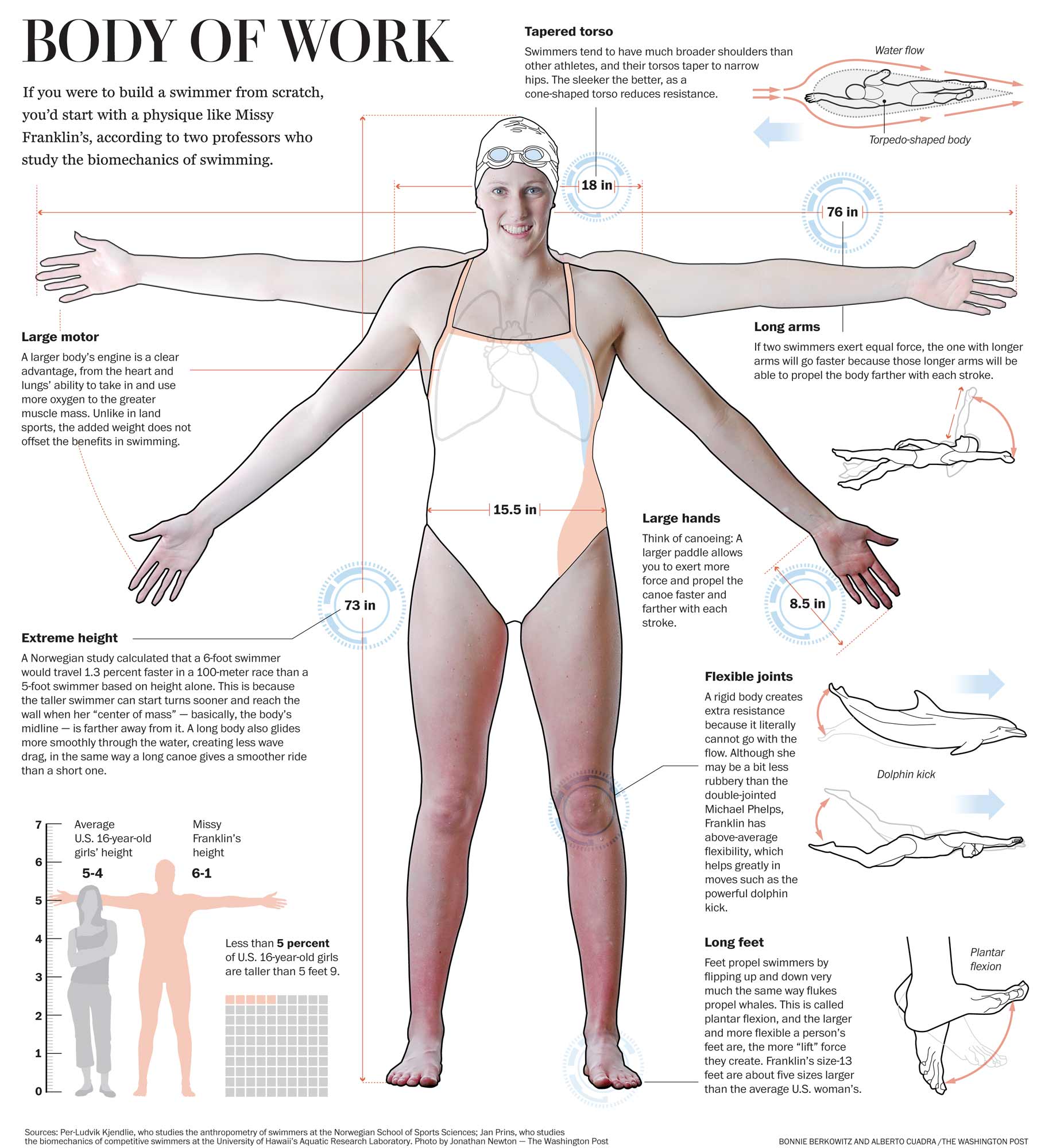This detailed diagram titled "Body of Work" focuses on the ideal physique for a swimmer, using Missy Franklin as the exemplar. The central image features a woman in a skin-tight swimsuit and swim cap, holding her arms out to the sides. Surrounding her are various annotations highlighting key physical attributes contributing to optimal swimming performance. The diagram emphasizes her extreme height of 6'1", which allows for faster turnarounds and a smoother glide through the water due to a longer body creating less wave drag. Her physique includes broad shoulders, a tapered and narrow torso, and long arms, all of which reduce water resistance and enhance propulsion. Visible notes also call out her large motor, referring to an effective heart and lung capacity that optimizes oxygen use and muscle mass, crucial for sustained energy. Highlighted too are her large hands, likened to paddles that increase force exertion with each stroke, and her long, flexible feet which function similarly to flippers, contributing to greater lift force during strokes. Missy Franklin's exceptional flexibility is noted, particularly in her joints, which reduces resistance and improves fluid motion in the water. The compilation of these physical traits outlines why Missy Franklin's body is archetypal for competitive swimming, showcasing how each feature—from height and muscle mass to limb length and flexibility—contributes to her excellence in the sport.